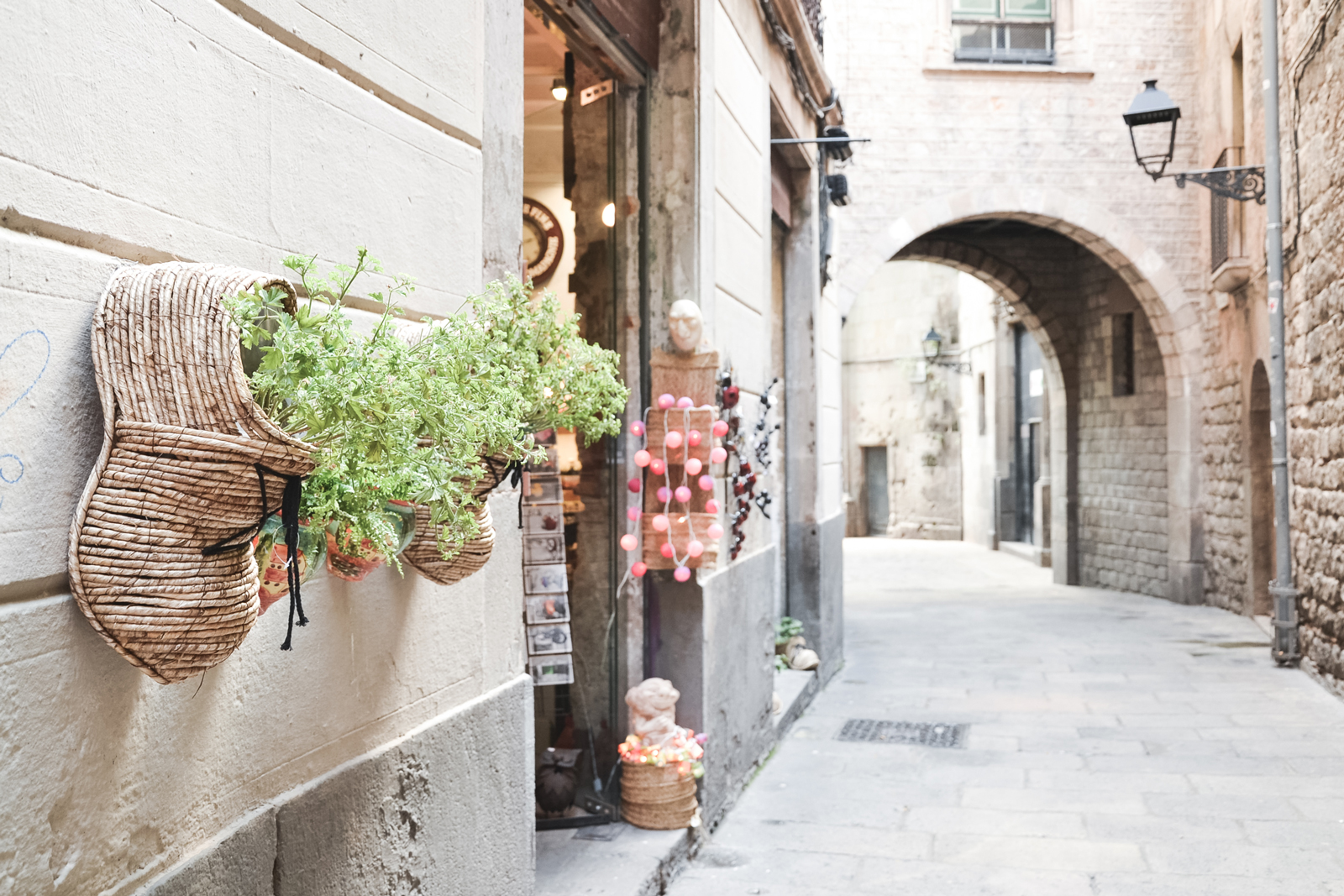The image captures a quaint European alleyway with a rustic charm. The pathway, paved with cobblestones, is flanked by brick buildings on either side, evoking an old-world ambiance. As you walk through this brightly lit alley, the scene unfolds like an open-air tunnel, with arches of buildings overhead. On the left, an inviting storefront displays postcards and festive paper lanterns, suggesting a vibrant local shop. A distinguished doorway, propped open by a small statue, hints at the entrance to this cozy establishment. Beautiful black lanterns line the right side, enhancing the alley's charm. Eye-catching decorative elements further add to the character: old-looking fabric shoes, appearing almost like they're crafted from brown paper or wood, are affixed to the walls, each acting as unique planters where thriving green plants sprout from the shoe openings. This inventive blend of natural beauty and rustic style gives the whole setting an enchanting, timeless feel.